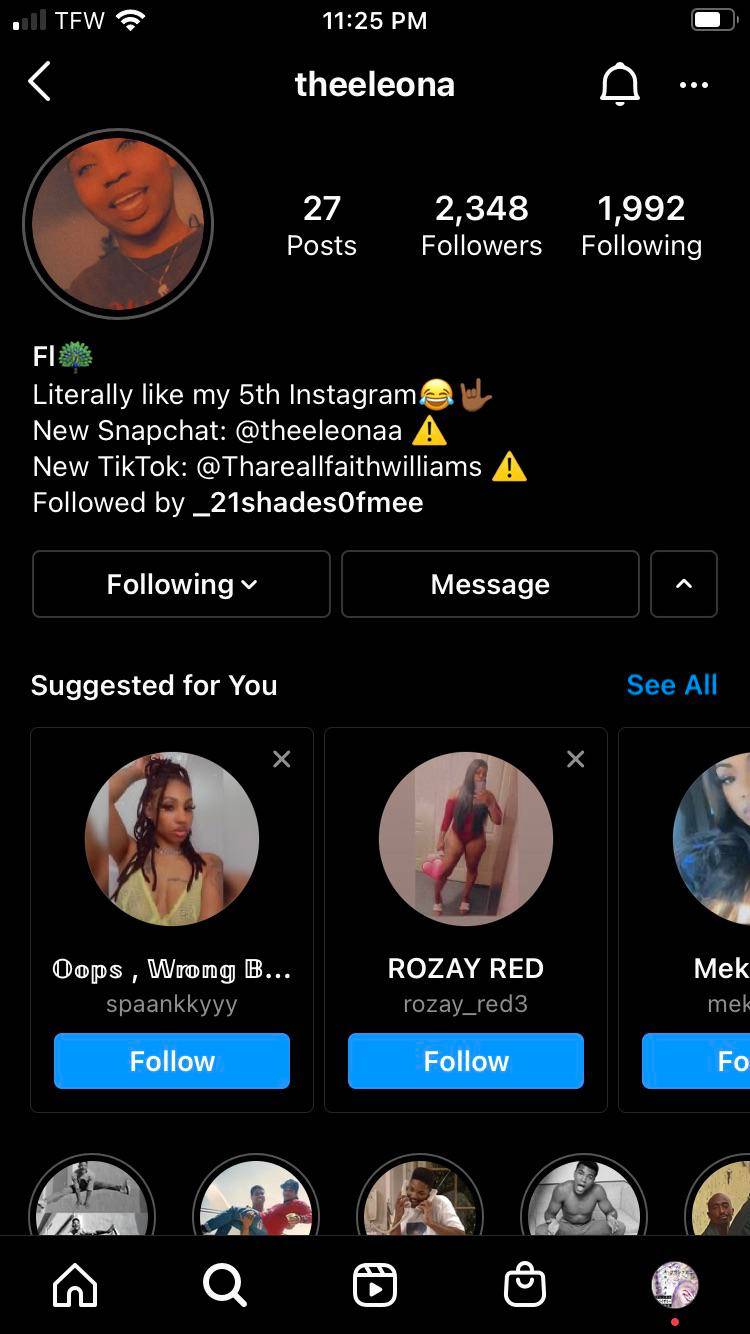This is a screenshot of a social media app viewed on a smartphone. The top of the screen displays various status icons, including a TFW icon with a full solid Wi-Fi signal, one out of four bars for cellular service, a battery meter showing approximately 75% charge, and a timestamp indicating 11:25 p.m.

In the middle portion, there is a profile header with the username "TheLeona" or possibly "TheLeonaA" (there is some ambiguity due to unclear audio). To the right of the username, there is a notification bell icon and a three-dot menu button. This interface bears some resemblance to Twitter, but the context provided suggests it might be Instagram.

Under the profile header, the statistics show "27 posts, 2,348 followers, and 1,992 following." Next to this, there is an "FL" notation with a tree icon. The bio section states, "literally like my fifth Instagram 😂🤙🐐," and further mentions, "new Snapchat: TheLeonaA," and "TikTok: @TheRealFaithWilliams," with a warning triangle icon.

The profile picture is visible and depicts an African-American woman who appears to be in her mid-twenties.

Below the profile information are options to "Follow" and "Message" the user. The "Suggested for You" section is immediately beneath, showing three African-American women with profile pictures and accompanying blue "Follow" buttons.

Lower still, there are icons representing notable African-American figures like Muhammad Ali, a young Will Smith, Tupac Shakur, and a few others, likely used as profile images for other individual profiles.

At the bottom of the screen, there are navigation buttons for home, search, play/video, shopping, and another unidentified profile or menu icon in the bottom-right corner.